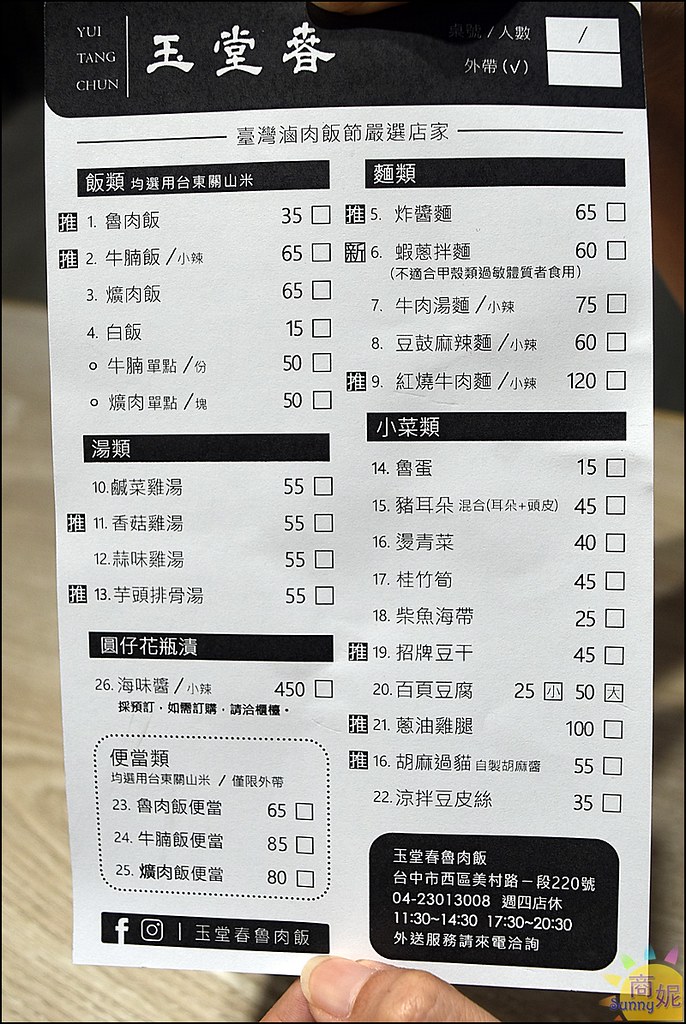The image depicts what appears to be a restaurant menu or form written in an Asian script, possibly Mandarin Chinese. At the very top, on the far left, there is a black box containing the name "Yu Teng Chun" along with three distinctive Asian characters in white print. Further to the right, there are two white letter boxes containing additional Asian script, likely placeholders for a date or other important information. The background of the photo is white with centrally aligned black lettering comprising numerous Asian characters. 

There are five unique black letter boxes lined up horizontally that each contain white Asian characters, with the traditional numeric labels 1, 2, 3, 4, and 5 underneath. Below each of these headings, there are corresponding checkboxes, suggesting an itemized menu with prices potentially in U.S. dollars. 

In the bottom left corner, there is a black box displaying social media icons for Facebook and Instagram. Meanwhile, in the bottom right corner, another black box contains white Asian script that likely lists dates, times of operation (1130-1430 and 1730-2030), and contact information, including a phone number (04-2301-3008). Notably, a circular emblem containing the word "Sunny" and two additional characters is also present in this area.

The photo captures the menu being held by a person with tan skin, prominently showing a thumb with a long fingernail at the bottom of the image.